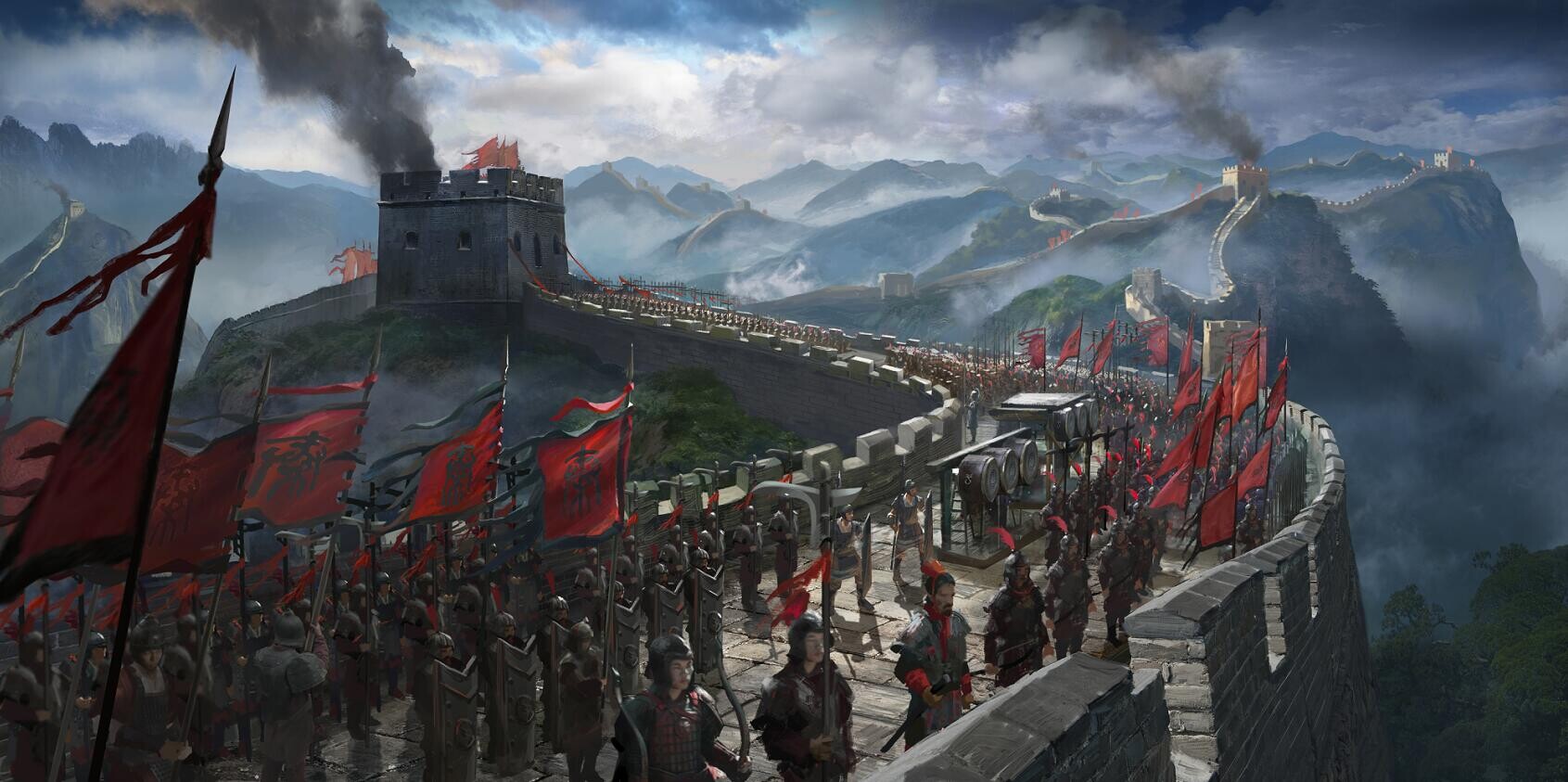The image depicts a dramatic medieval scene, seemingly captured from a movie, showcasing the Great Wall of China teeming with hundreds of soldiers in uniform. The wall, tall and imposing, curves gracefully to the left and extends into the distance, nestled among rugged mountains. Central to the composition, the soldiers, adorned in gray armor with striking red accents and hats, stand in disciplined rows along the wall, which is under siege. They wield bows and arrows and display numerous tall flags with red banners bearing black Chinese characters. Smoke and fire emerge ominously from multiple towers along the wall, hinting at ongoing battles. The sky above is a tumultuous mix of blue, gray, and white clouds, intensifying the scene's tension. The flags, central to the image, flutter defiantly against the backdrop of the fortress engulfed in smoke and flames, while the soldiers’ stern gazes are directed off to the right, perpetuating the sense of impending combat.